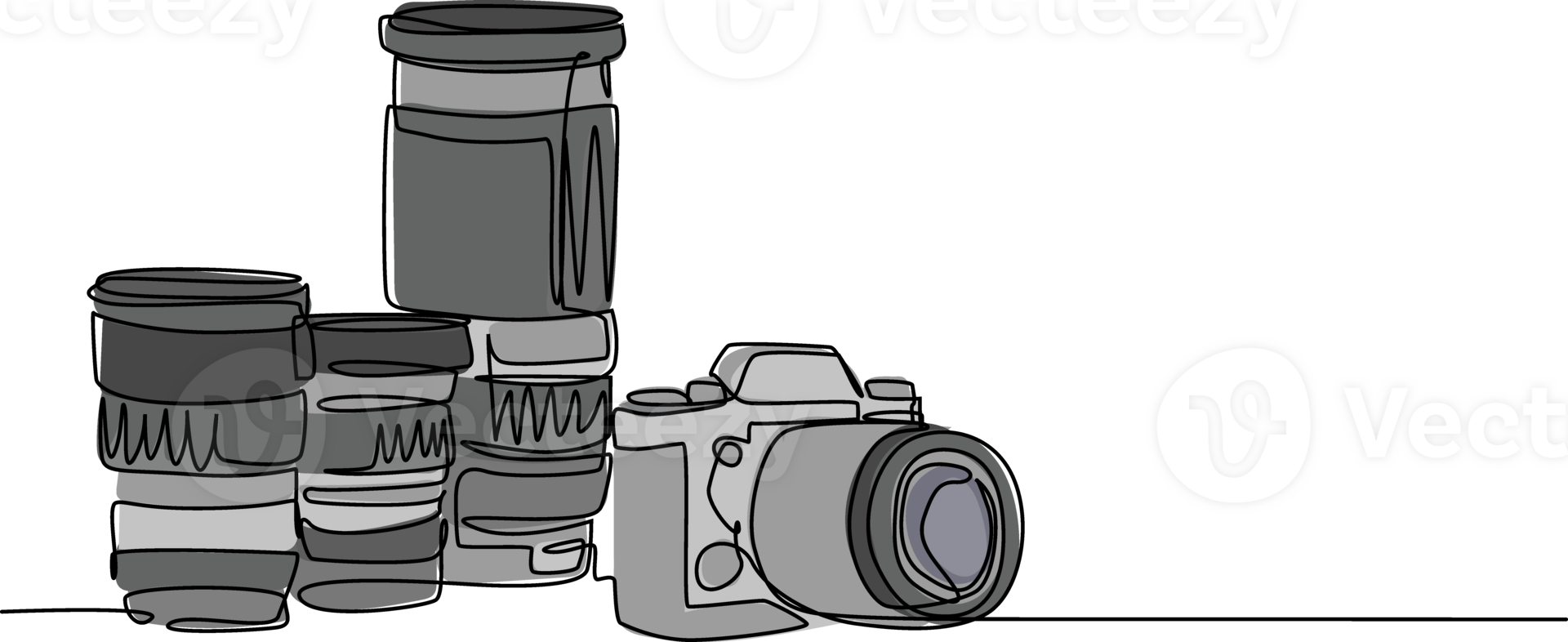The image features a detailed black and white drawing on a white background, subtly marked with a faint black and white "Vecteezy" watermark, indicating its source. The central object is a gray 35mm camera with a lens attached, rendered in detailed black outlines. The camera points towards the right and sits upon a thick black line, indicating a surface. To the left of the camera, four additional interchangeable lenses are depicted. There are three lenses arranged at the bottom, with the first being the tallest, and another lens similarly sized to the shorter ones stacked above them. All elements in the drawing, including the camera and lenses, are shaded in various tones of gray, giving a cohesive monochromatic aesthetic that appears to be meticulously hand-drawn and possibly digitally refined.